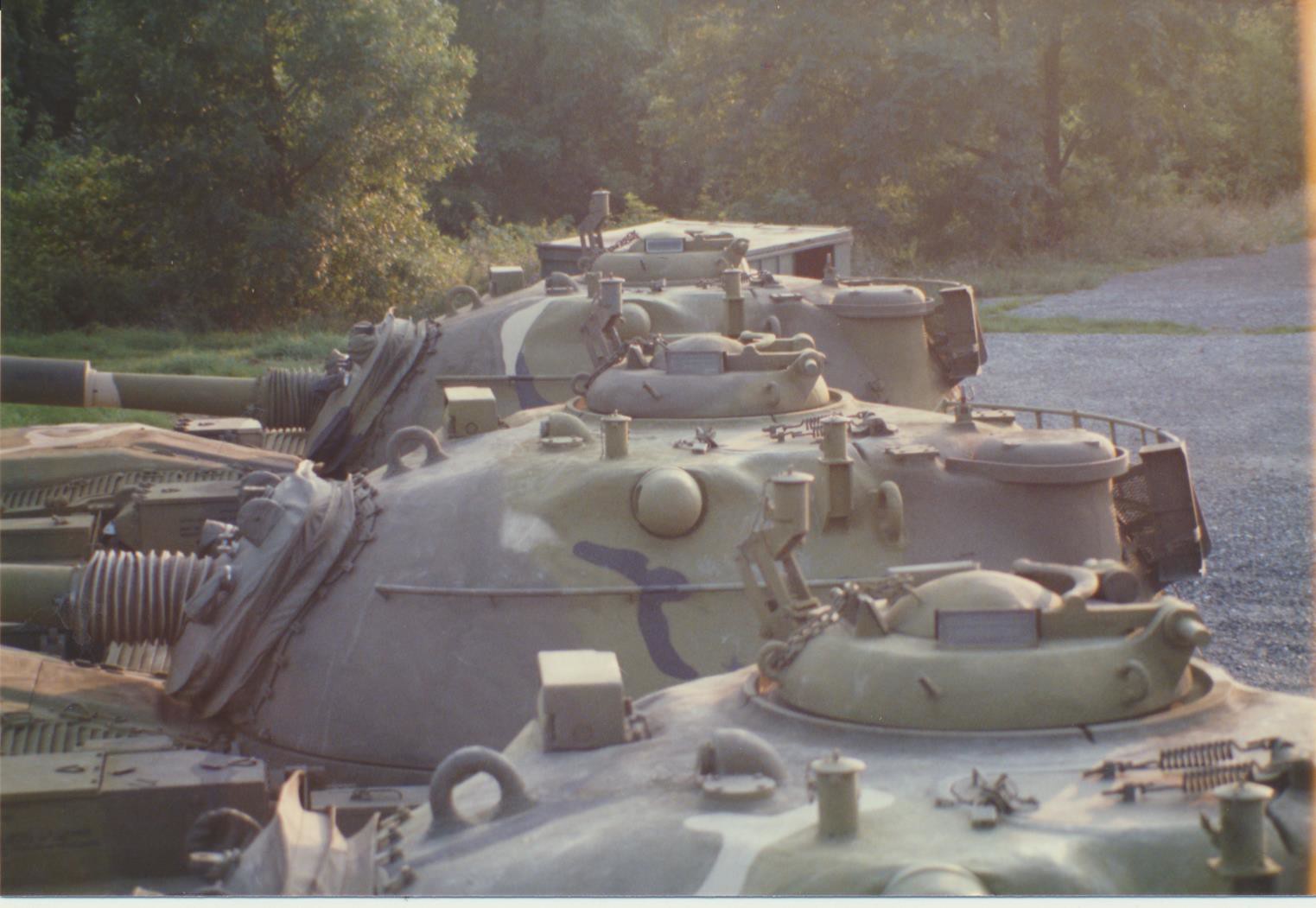This color photograph, taken outdoors in natural lighting, depicts a row of three large, grey industrial or military objects, possibly tanks, lined horizontally on a somewhat blue, tarmacked surface intersected by a sliver of grass in the left corner. The primary objects are distinguished by their semi-circular, curved shapes and a camouflage pattern of drab brown and green. They feature round protrusions, cylindrical structures, and railings around the front of the middle and back sections, with large tubes connected towards the rear. Visible from a level equal to their tops, the equipment fills the lower part of the frame with varying degrees of visibility — the front one almost completely, the middle one prominently, and the back one moderately. In the background, to the left and center, lies a dense wooded area illuminated by sunlight, suggesting an autumn setting with trees displaying yellowish hues. A gravel road is faintly visible on the right side, adding to the outdoor scenery's muted, overcast ambiance.